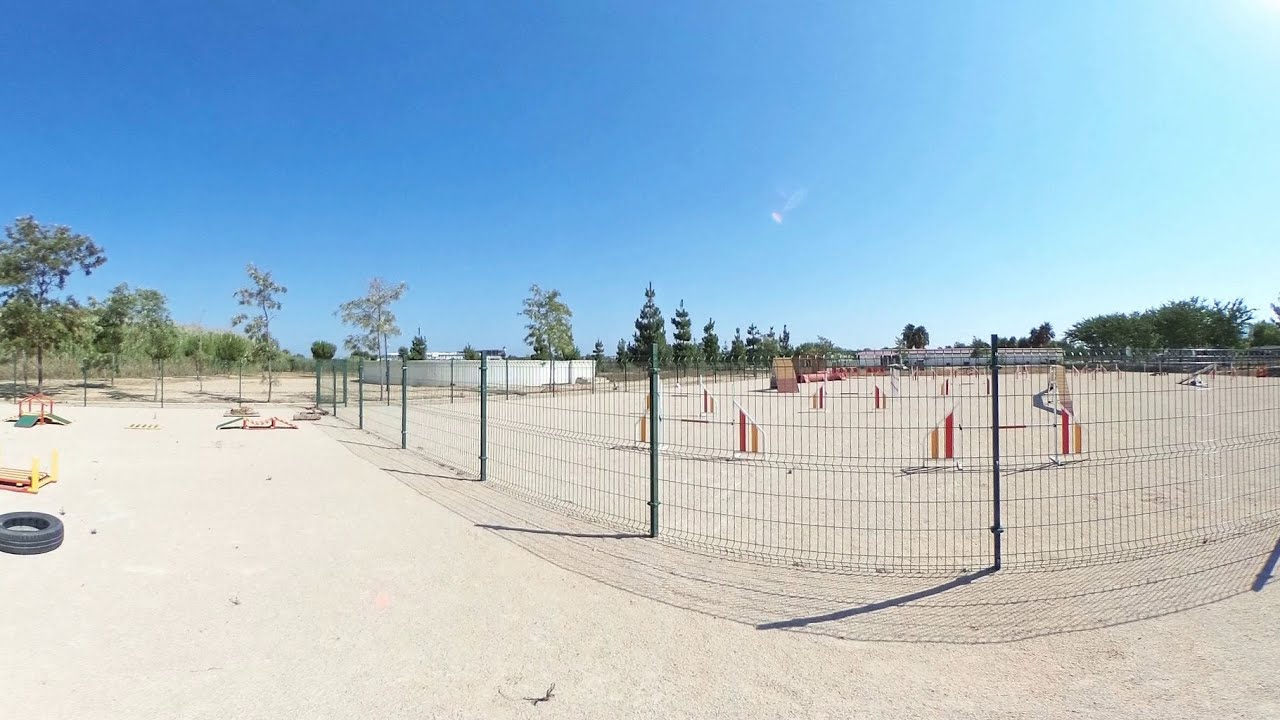This photograph captures a spacious park surrounded by a uniquely designed fence with small squares, approximately three feet high. The area within the fence appears to be split into two sections: a sandy zone on the left and a more structured obstacle course on the right. The right side features elements suggesting possible uses for activities like go-karting or dog competitions; noticeable structures include red and yellow columns, a ramp, and what seems to be a seesaw. Scattered around the area are various toys and items, including a black tire. Further in the distance, beyond the fence, stands a line of taller pine trees and additional sparse trees dotting the landscape. The background is marked by a blue sky, indicating a clear, sunny day with no visible clouds. There are no people present in the photograph, and it lacks identifiable markers such as a date, time, or specific location.